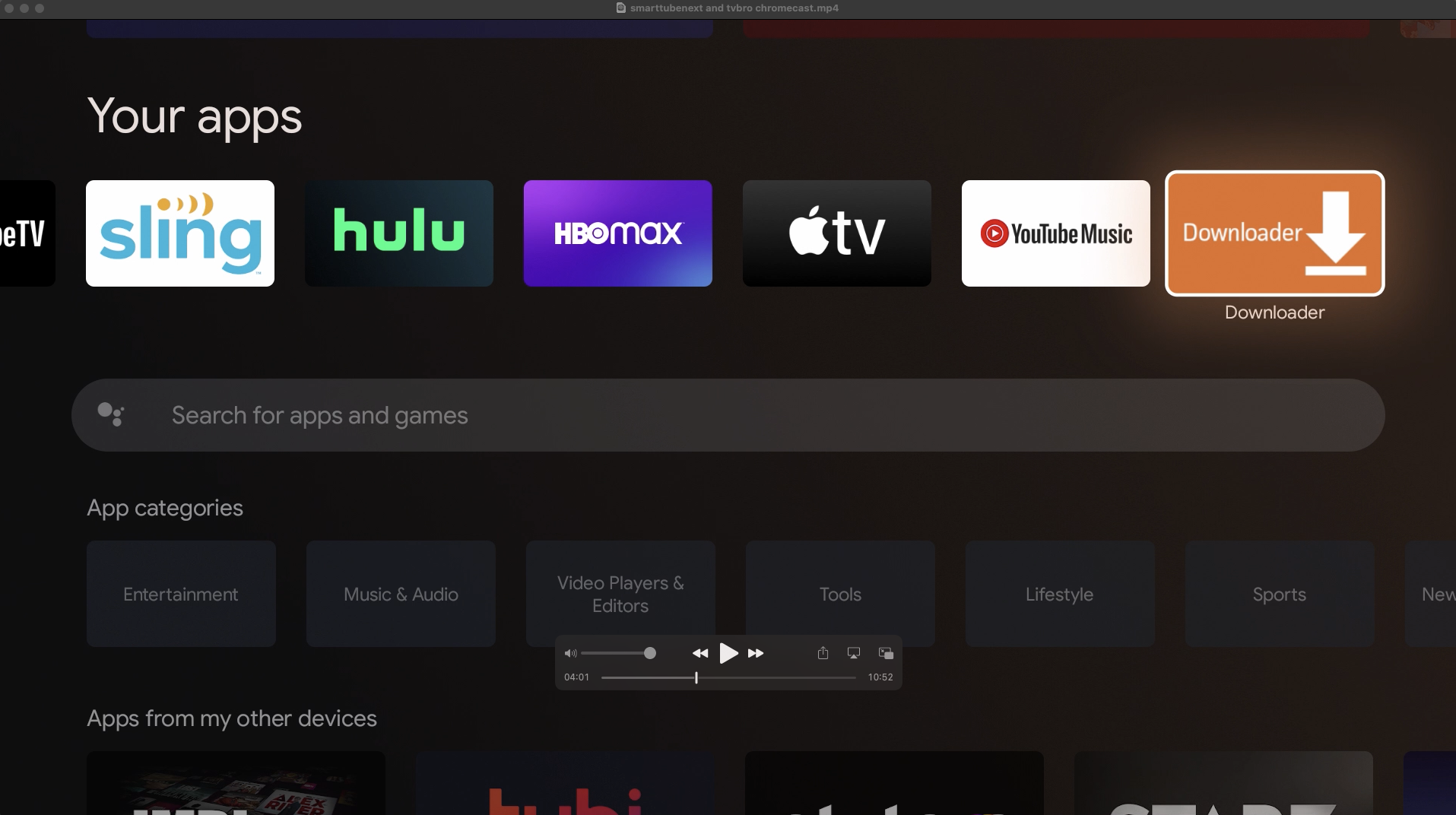The image depicts a dark black screen showcasing a range of notable apps, organized from left to right. Here's a detailed breakdown:

- **Sling**: The first app on the left.
- **Hulu**: Positioned next, featuring its signature green and black typography.
- **HBO Max**: This app is represented by a white logo against a plain blue background.
- **Apple TV**: Following in the lineup with a white apple logo set against a stark black background.
- **YouTube Music**: Nestled beside Apple TV, a white box adorned with a red logo resembling a Target emblem, creating a sharp contrast.
- **Downloader**: The last app on the right, characterized by its bright orange rectangular icon. The icon includes a white arrow pointing to a bar, indicating a download function.

Below these primary app icons, various categories are available for quick access, catering to different user interests. These categories include:

- Entertainment
- Music & Audio
- Video Players & Editors
- Tools
- Lifestyle
- Sports

This interface appears designed for individuals who prioritize practicality and convenience, possibly for those who lack time to engage deeply with traditional media. A prominent oblong search bar in the middle of the screen invites users to "Search for apps and games," further underscoring the emphasis on ease of access and quick navigation.